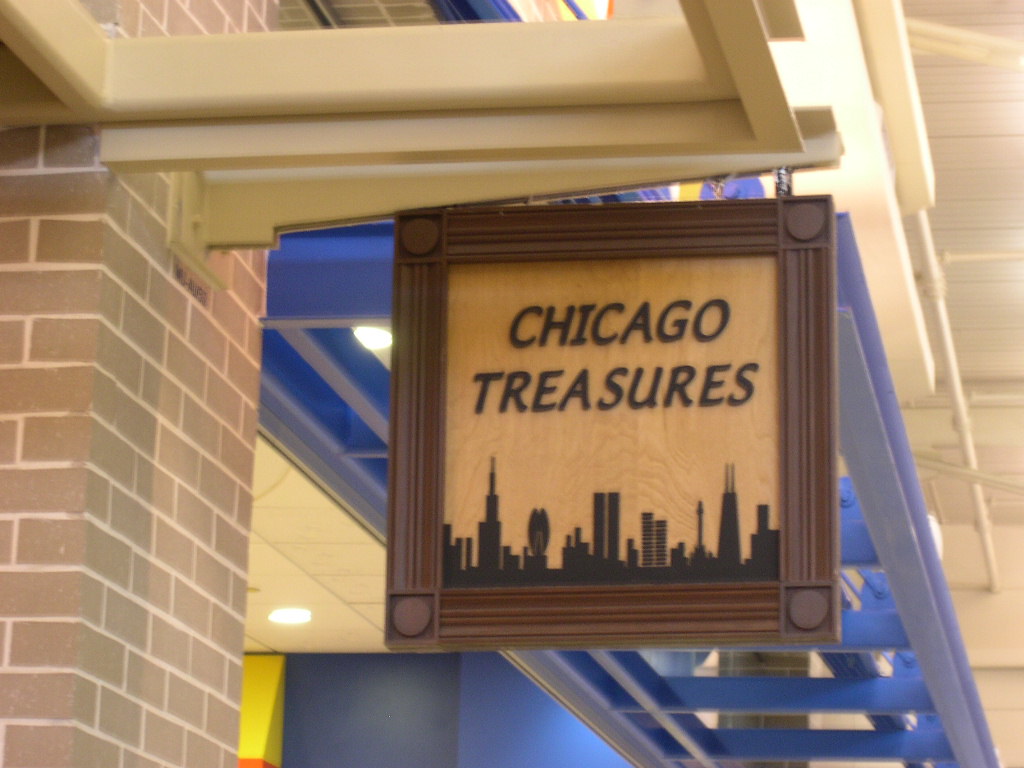A close-up image showcases a small, square wooden sign hanging horizontally from a tan metal awning attached to a brick building. The sign, which serves as an eye-catching storefront indicator, features a light-colored plywood background with the words "Chicago Treasures" emblazoned in brown. At the bottom of the sign, a black silhouette of a cityscape with towering skyscrapers adds a unique decorative touch. Encasing the sign is a brown frame with detailed lines and dots at each corner, reminiscent of a picture frame. To the left of the sign, the building's brick facade is visible, providing a textured contrast. In the background, a blue metal awning from the adjacent business peeks into view, adding a splash of color to the composition. The bottom center of the photo reveals more of the neighboring blue building, subtly completing the urban setting.